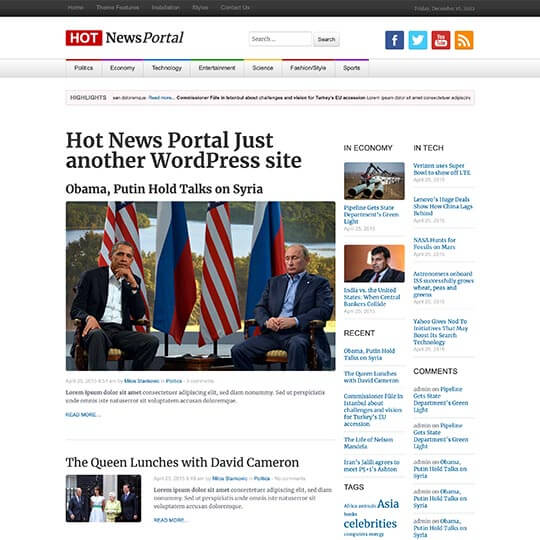In the image of the "Hot News Portal" website, the title "Hot News Portal" is prominently displayed, with the word "Hot" in bold red letters and "News Portal" in bold white uppercase letters. Below this title, a search bar and several social media icons for Facebook, Twitter, YouTube, and sharing are neatly aligned. 

Under this section, the website categorizes its content into various sections, including Police, Politics, Economy, Technology, Entertainment, Science, Fashion, Style, and Sports, allowing users to easily access their topics of interest by clicking the respective categories. 

A highlights bar, which features some highlighted text, separates the categories from the main content beneath it. The primary headline beneath this bar reads "Hot News Portal - Just Another WordPress Site." Below this, there is a lead story featuring an image of Barack Obama and Vladimir Putin engaged in serious discussion about Syria. In the image, Obama, seated on the left, rests his left arm on his chin, while Putin, seated on the right, sits upright with both arms on his lap and looks downward. The American and Russian flags are displayed behind them.

Following this main article, another headline reads, "The Queen Launches with David Cameron." Adjacent to the main articles, the right-hand column displays various sections of content, including Economy and Technology, providing a comprehensive overview of recent news updates.